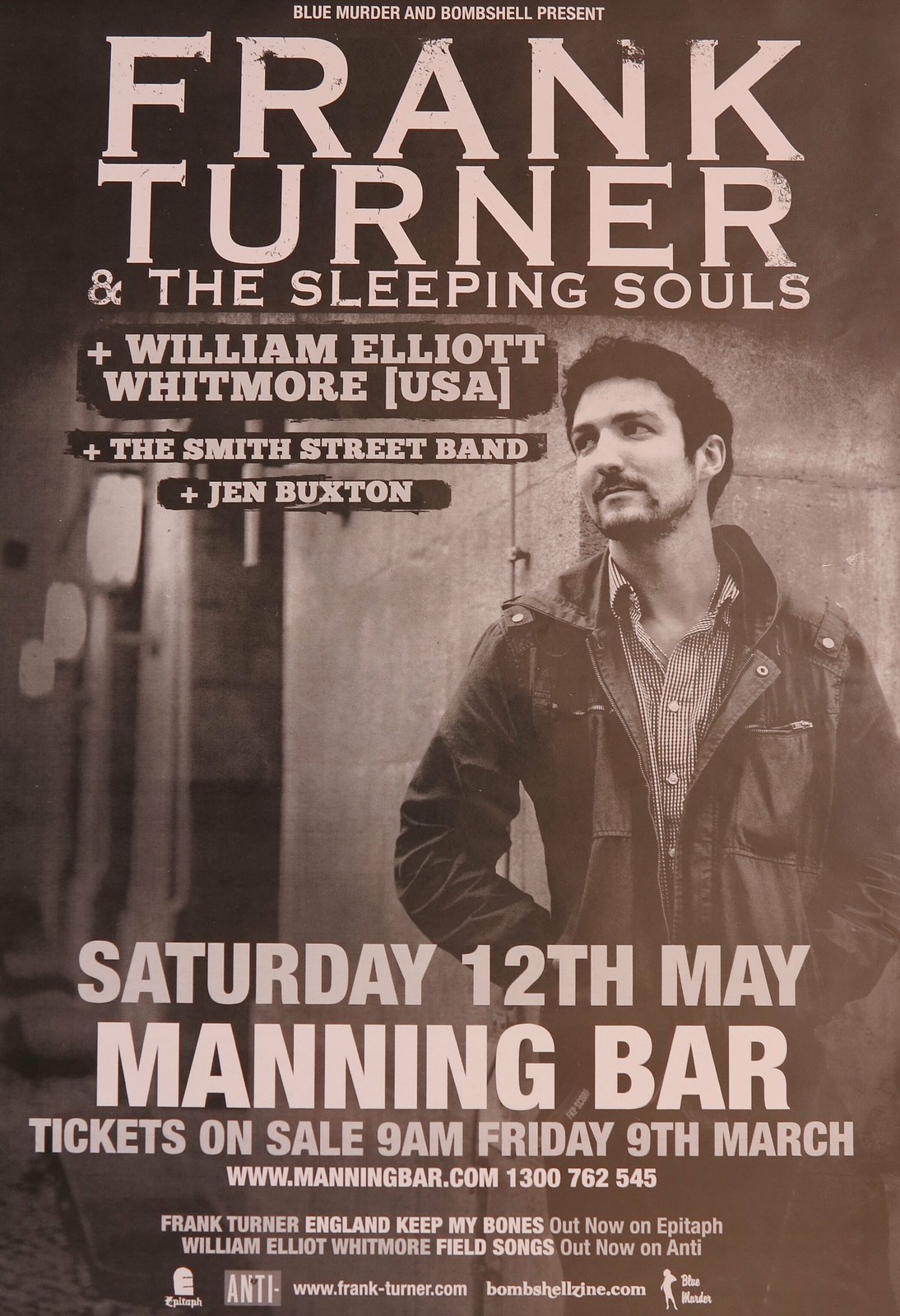This is a detailed description of a vintage-style concert poster for Frank Turner and the Sleeping Souls. The poster features a black-and-white image with a brownish sepia tone tint. At the top of the poster, "Blue Murder and Bombshell Present" is prominently displayed, followed by the name "Frank Turner and the Sleeping Souls" in large lettering. Supporting acts include William Elliot Whitmore from the USA, The Smith Street Band, and Jen Buxton. The event is scheduled for Saturday, May 12th, at the Manning Bar.

The photograph on the poster showcases a young white man around 20 years old, presumably Frank Turner. He has dark hair and light facial hair, wears a leather jacket over a button-down shirt, and leans against a concrete wall, looking off into the distance to the left. The image evokes a moody, contemplative atmosphere.

Further details include that tickets go on sale at 9 a.m. on Friday, March 9th. The poster also provides the website www.manningbar.com for purchasing tickets. Based on context, it seems this event is taking place in England.